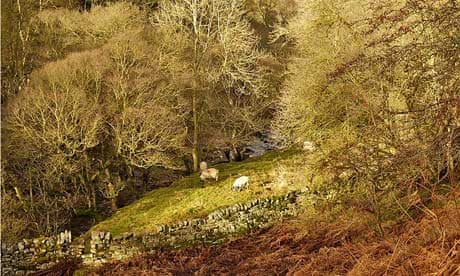The image depicts a detailed landscape, resembling a painting set in early spring. The scene is dominated by bare trees with a patch of lush green amidst predominantly brown grass. On the right-hand side, a large, leafless tree stands prominent. The sun, unseen but inferred from the lighting, shines from the top right corner, casting light across the field.

In the middle ground, a small hill slopes gently down to what appears to be a stream, hinted at by a crevice at the bottom. The landscape transitions from an overgrown brush in the foreground, characterized by patches of red foliage, to a greener pasture, eventually meeting a stone wall that stretches across the frame left to right.

Behind the wall, two small animals—possibly sheep, goats, or even ducklings—graze peacefully, reinforcing the tranquil setting. These animals seem to be raised for their wool or are young, adding an element of life to the overgrown wild area. The background is filled with more barren trees, establishing a forest that stretches across the horizon, completing the serene, early spring depiction.